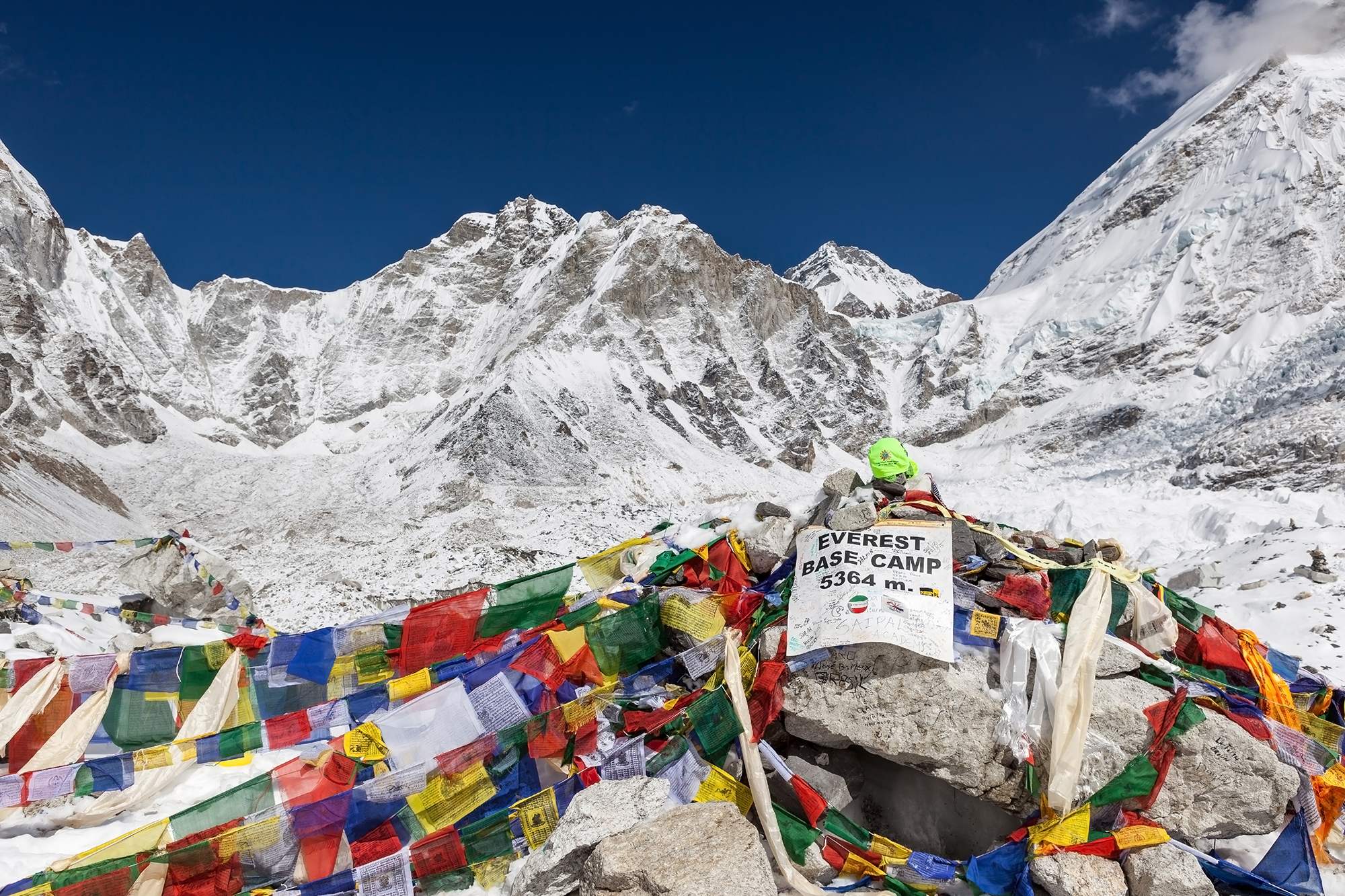The image is a stunning outdoor photograph taken at Everest Base Camp during the daytime. The rectangular photograph measures approximately six inches wide by four inches high. It features the majestic peaks of the snow-capped mountains on both the left and right sides, with small patches of brown rock peeking through. In the bottom foreground, there is a mound of light-colored rocks adorned with a variety of small, colorful flags in red, green, blue, and yellow, as well as pieces of paper. At the very center of the image, a white fabric or paper sheet prominently displays the text "Everest Base Camp 5364 meters" in black print, surrounded by numerous signatures from climbers and tourists. Above the mountains, the sky is a vibrant blue with only a few clouds, one of which is visible on the right side. The scene is devoid of plants or trees, emphasizing the snow-covered, rugged terrain. The colorful flags draped over the rocks add a traditional and cultural touch, possibly representing Tibetan prayer flags or those from Nepal.